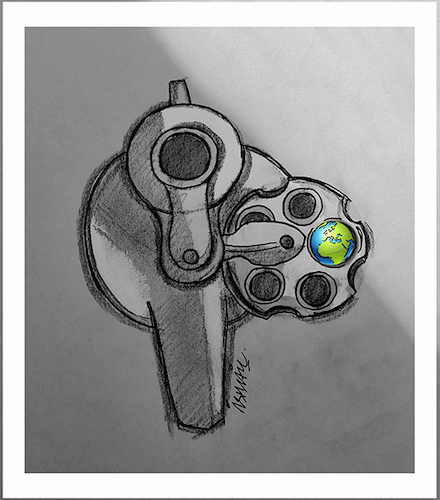This detailed hand sketch of a revolver features the side chamber pulled out and open, revealing five circular chambers. Four of these chambers are hollow and colored in black, while one showcases a colored drawing of the globe, with green landmasses and blue oceans, focusing on Europe and Africa. The gun is oriented as if pointing directly at the viewer, providing a direct view down its barrel, which is shaded in dark black. The revolver itself is meticulously drawn in varying shades of gray, from light to dark, with a striking contrast against the charcoal black background. The background features gradient shading, transitioning from a lighter gray in the top right corner to a darker gray covering the bottom two-thirds. The image is framed with white trim around its edges. Below the revolver, near the bottom, is a scribbled signature of the artist, though it is indistinct and difficult to decipher. The overall composition highlights a stark, almost confrontational perspective, emphasizing the detailed craftsmanship of the drawing.